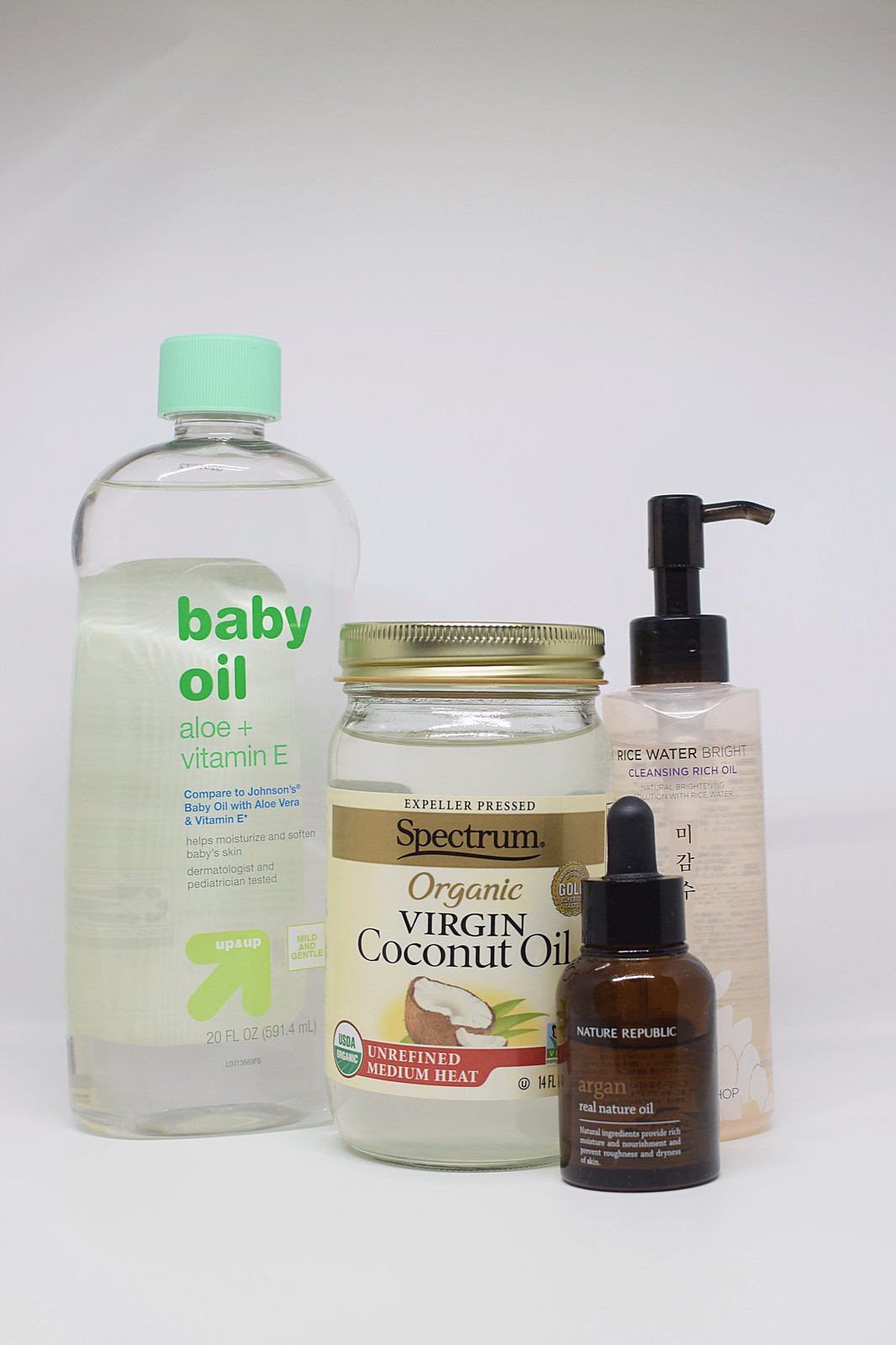A minimalist bathroom shelf displays a collection of personal care products set against an all-white backdrop, blending the surface and wall into a seamless, nondescript expanse. On the far left stands a clear bottle of Up & Up brand baby oil, identifiable by its pale green cap and green-and-blue product details. The bottle features aloe and vitamin E prominently on its label, with the Up & Up logo in a light green color.

Centrally positioned, a jar of Spectrum Organic Virgin Coconut Oil catches the eye. The jar, which resembles a mason jar, is topped with a brass-colored lid and boasts various certifications, including a red strip indicating it’s unrefined and suited for medium heat.

To the right of the coconut oil is a smaller brown glass vial with a dropper, presumably from Nature Republic. Though the white text is somewhat difficult to read, the jar likely contains argan oil. The vial measures about two-thirds the height of the adjoining coconut oil jar.

Behind and slightly to the right of this vial is another intriguing item, a clear plastic pump bottle with Asian text, likely denoting it as a rice water cleansing oil. The black dispensing pump of this bottle stands just over an inch higher than the coconut oil jar, giving a varied height aesthetic to the neatly arranged shelf.